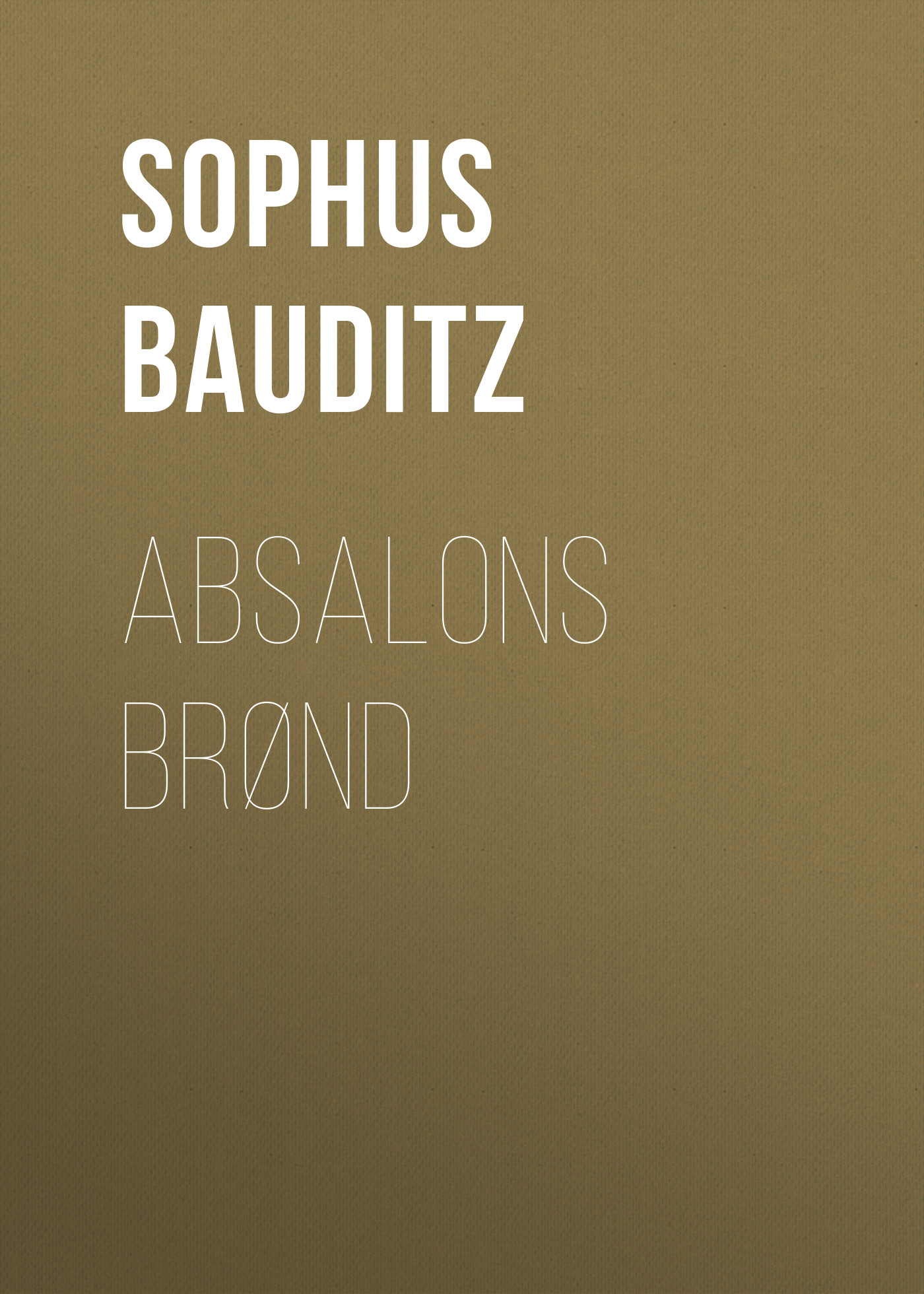The image depicts a vertical rectangle with a deep olive drab bronze gradient, slightly lighter at the top. In the upper left portion, two bold lines of all-caps white text read "SOPHUS" and "BAUDITZ." Below, in a thinner font, appear the words "ABSALONS" and "BRØND." The background is a solid, metallic gold color, suggesting the appearance of an old book cover. The text and color palette dominate the image, with no other graphics or objects present.